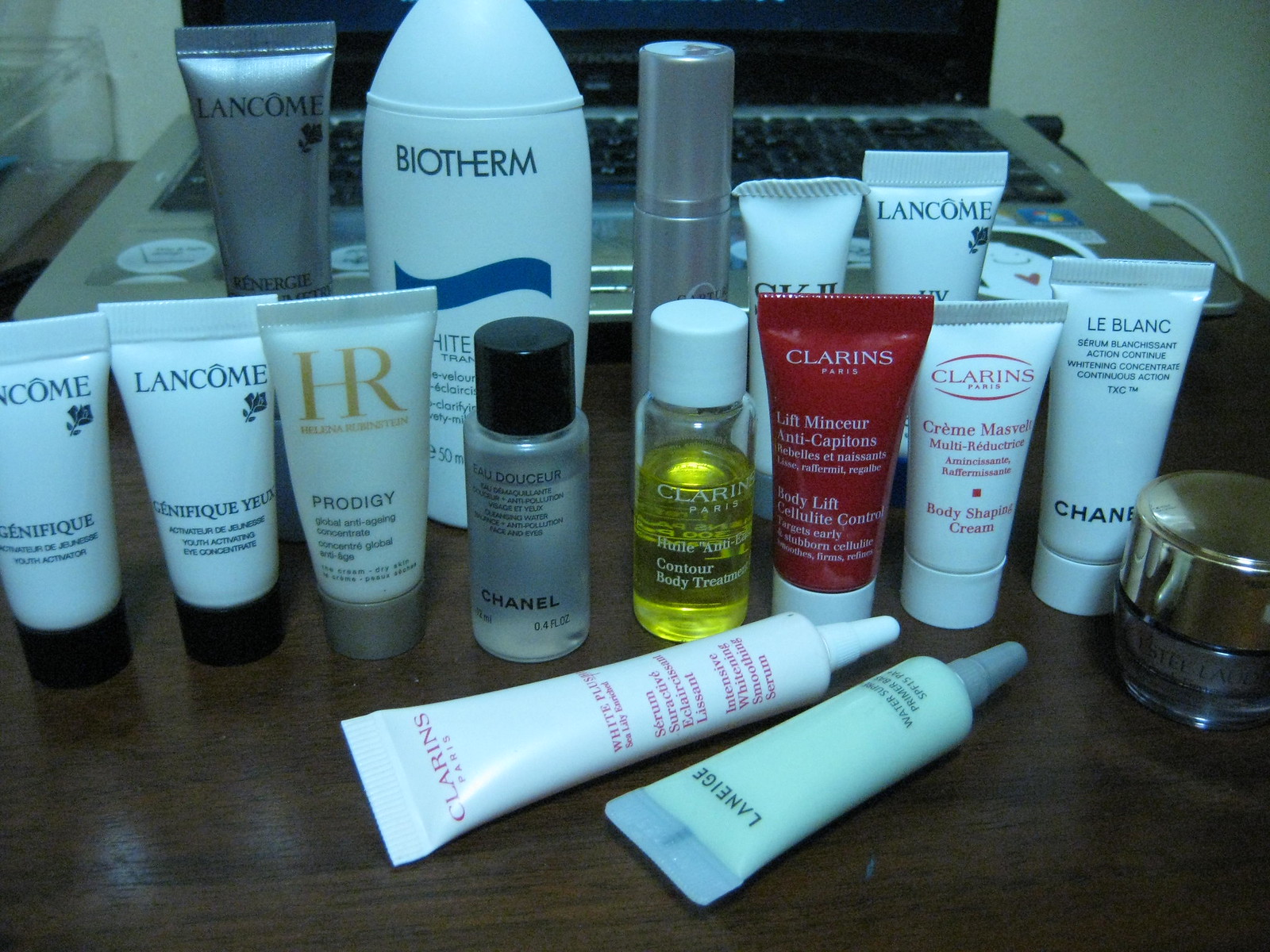The image showcases a close-up view of various beauty products neatly arranged on a deep walnut-colored wooden desk. An open laptop is positioned behind the assortment of beauty products, indicating a workspace that seamlessly blends productivity and self-care. From left to right, the collection begins with two white plastic tubes of LAMCOM products, featuring black caps. Adjacent to the LAMCOM items is a Prodigy product in an off-white tube with a grey cap. Behind the Prodigy product, a silver-grey LAMCOM tube adds a touch of elegance to the lineup. Positioned next to the silver-grey tube is a large bottle of BALTEM. In the foreground, a small clear bottle prominently displays the Chanel brand, adding a luxurious flair. Additionally, products from Clarence and Le Blanc complete the diverse array of premium beauty items, showcasing a variety of skincare choices.